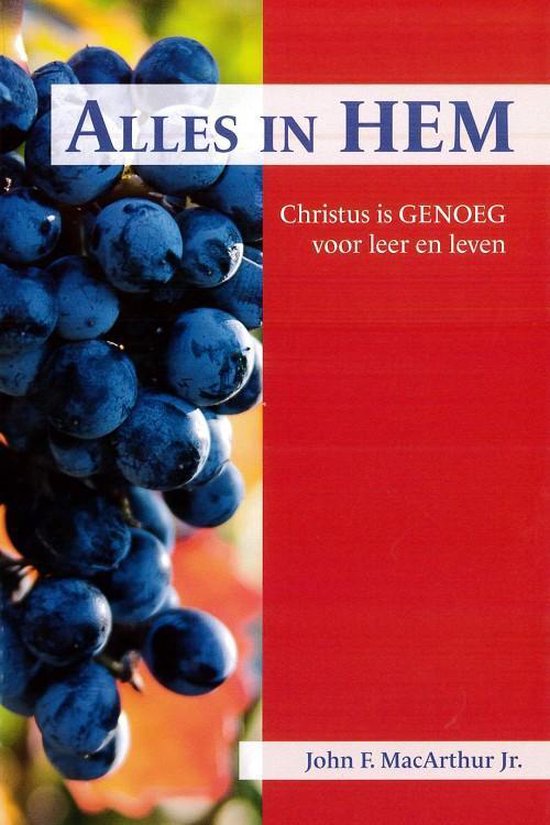This is the cover of a book titled "L.A.'s and Him" by John F. McArthur Jr. The design is split into two vertical sections. The left side features a close-up image of vividly blue blueberries, some of which are lighter or slightly darker, connected in clumps with a blurred green and orange background. On the right side, there is a solid red background with white text in what appears to be Dutch, reading "Christus is Gina A. Forley and Aidan Levin." The title "L.A.'s and Him" is centrally positioned at the top of the cover in blue font, spanning both sections. At the very bottom, in a rectangular peach-colored box, the author's name, John F. McArthur Jr., is displayed in blue text.